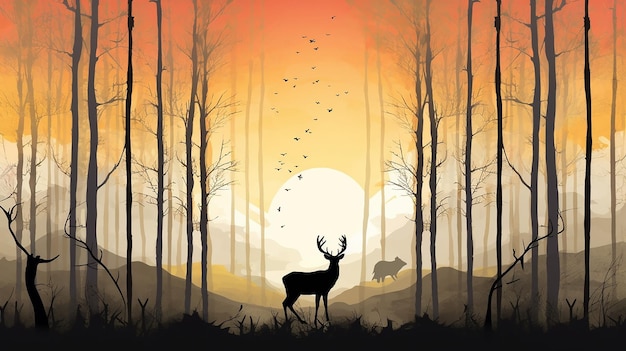The image is an AI-generated illustration depicting a mysterious and majestic forest scene at sunset. The background transitions from a deep orange to a lighter orange and then to a yellow, resembling a scenic ombre sunset. A white sun sets in the center of this gradient. Silhouetted in the foreground is a black deer with prominent antlers. Next to the deer, there is a lighter-colored animal, possibly a bear or pig, positioned further back. On either side of the image, tall, spindly trees without leaves stretch upwards, adding a somewhat eerie vibe. Dark vegetation sprawls at the feet of the deer, anchoring the foreground. Scattered throughout the sky are small, faint black birds flying in the distance, enhancing the sense of depth and liveliness in this burnt and skeletal forest landscape.